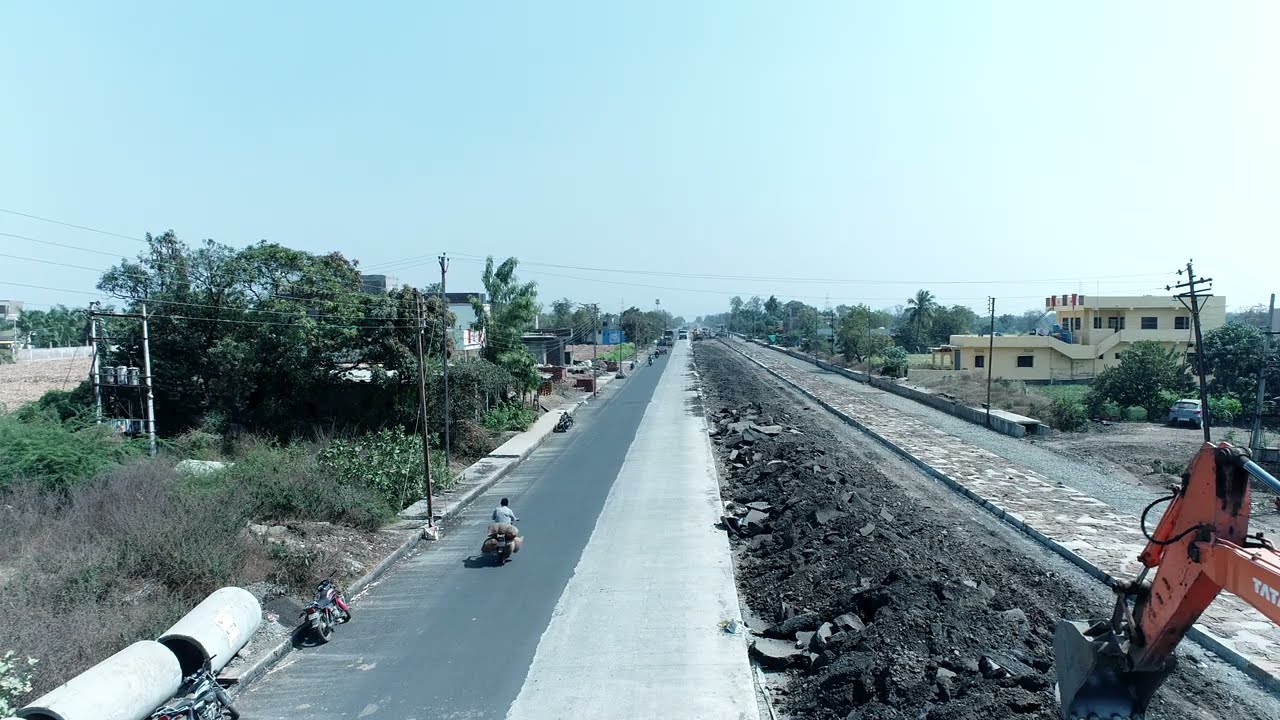In an urban setting, a road construction project is well underway, dividing the image into distinct segments. Straight through the center, two roads run parallel. On the left, a completed dark gray road wide enough for two cars hosts a single motorcyclist driving in the middle, clad in white without a helmet. Flanking this finished road on its left are various green and brown shrubs and vegetation, intermittently interrupted by power lines stretching through the scenery. Adjacent to this is a stark contrast: a partially demolished road section with broken concrete, where an orange and black excavator diligently digs up the surface in the bottom right corner. The area exudes a sense of neglect and ongoing transformation, amplified by additional power lines visible on both sides and complemented by a cream or light yellow multi-storied building in the right background. White text overlays parts of the image, further highlighting the contrast between the areas.